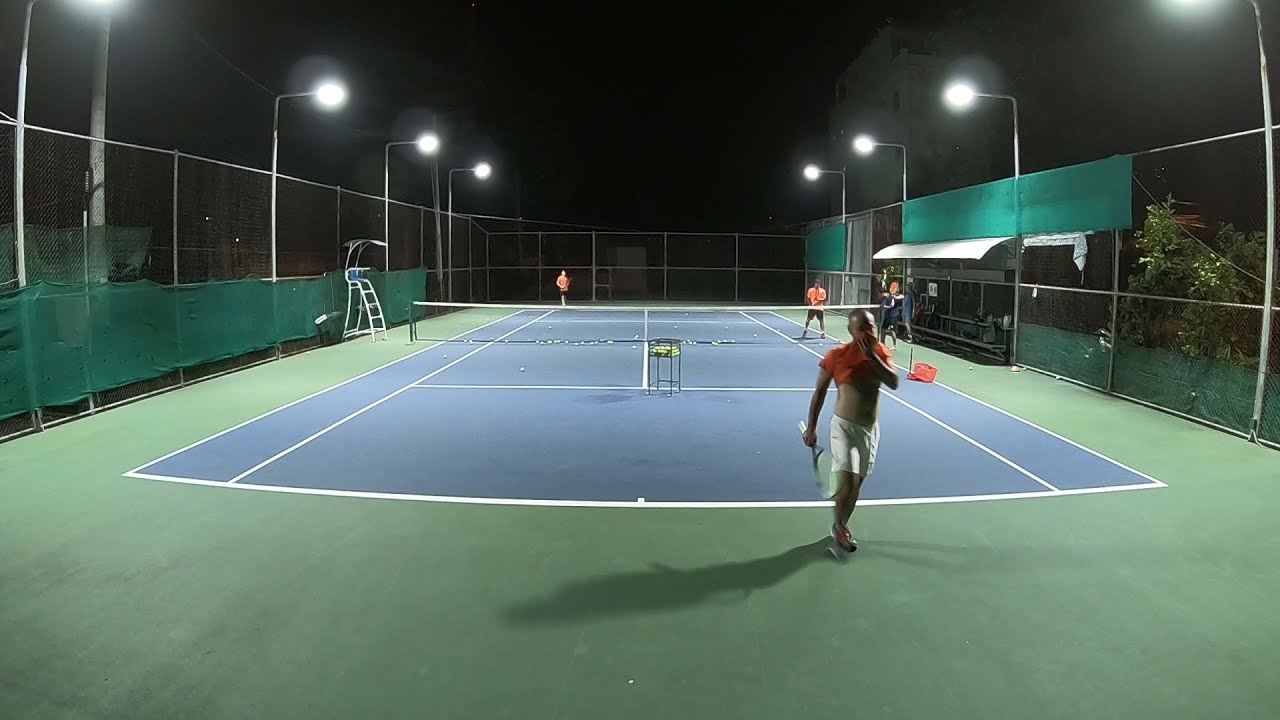This is a detailed nighttime photo of an illuminated outdoor tennis court. The sky is completely black, enhancing the bright lighting provided by eight streetlights surrounding the court. The court features a blue playing surface with white striping, while the out-of-bounds areas are green. Surrounding the court are silver fences, with green screen padding along their bottoms.

In the foreground, slightly right of center, a man wearing an orange shirt and white shorts walks towards the camera, holding a tennis racket. He appears to be wiping sweat off his face with his shirt. On his side of the court, there is a container filled with tennis balls. Behind the man, on the other side of the net, stand his two opponents, both dressed in orange tops and black shorts. To the left of the net is a chair typically reserved for a referee. The image captures the intensity and setting of an evening tennis match with clarity and detail.